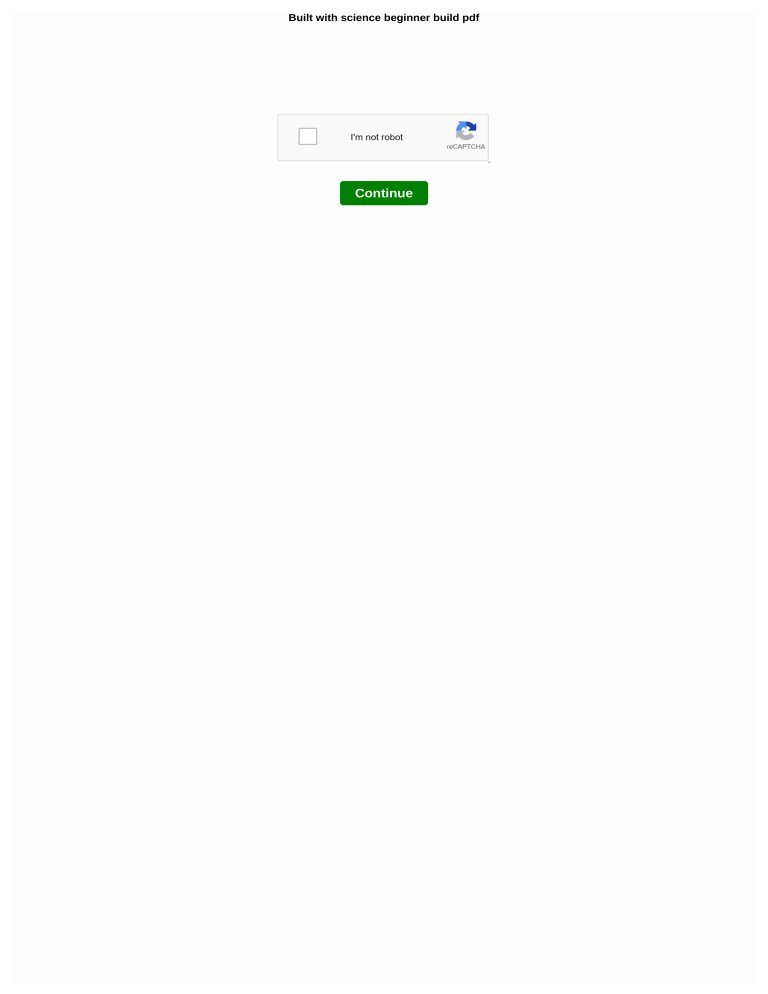This image features a minimalistic design with a predominantly white background. At the top, there is a small black font text that reads, "Built with Science Beginner Build PDF." Below this text lies a blue rectangular box that contains a smaller white checkbox labeled, "I'm not a robot," accompanied by a blue and gray arrow icon symbolizing CAPTCHA verification. Positioned underneath this is a prominent green button with the word "Continue" written on it. The overall composition is straightforward, focusing prominently on the CAPTCHA verification process and the action button, set against the simple white backdrop.